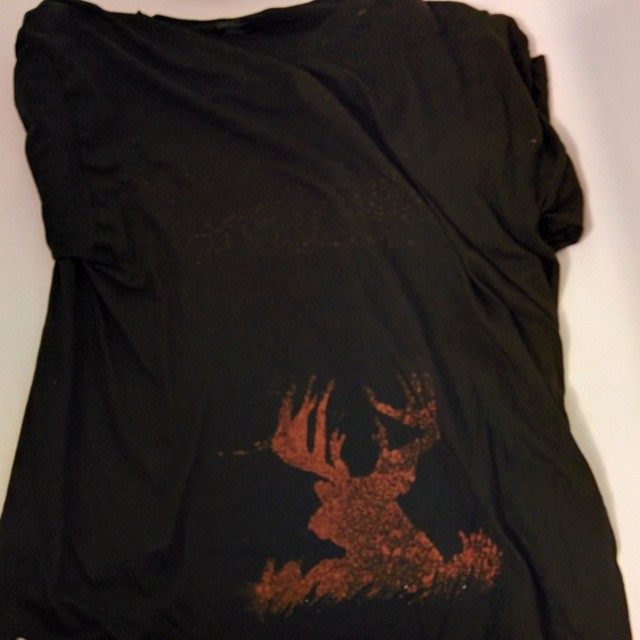This is a photograph of a crumpled, sleeveless t-shirt, which appears either extremely dark brown or black, possibly faded and old. The backdrop of the image is predominantly light purple with white light illuminating the right-hand side. The focus is on the bottom part of the t-shirt, where an intricate orange design illustrates a deer. The deer's head is outlined with antlers, an ear, and a partial face visible, suggesting it is crouching in a patch of grass. The design, which also incorporates brown, especially at the bottom, gives the impression of a moose or deer nestled in grass. The shirt itself has areas that seem extra faded, almost as if bleached, adding to its worn look. Shadows from the t-shirt are cast onto the background, adding depth to the image.